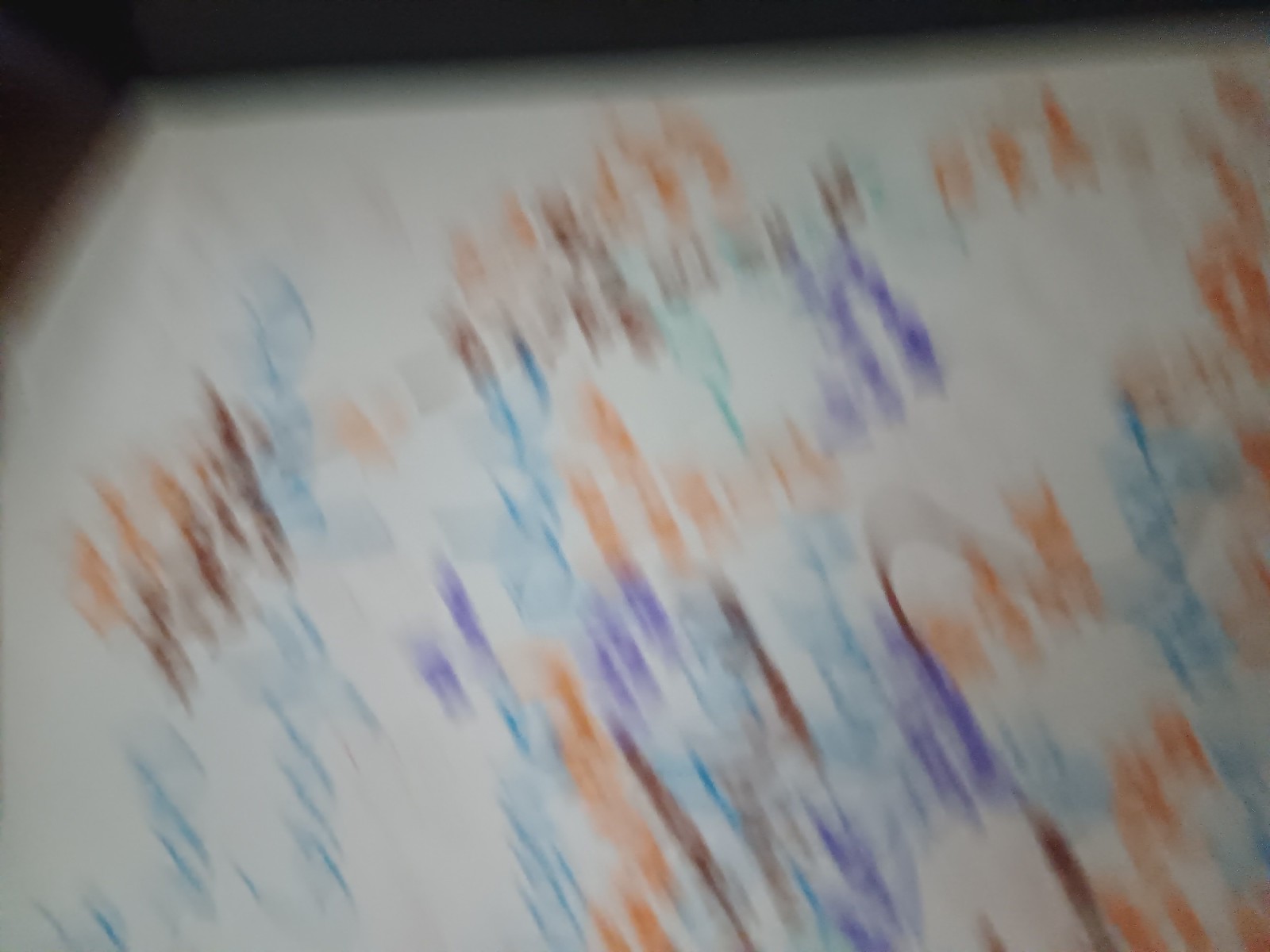A highly blurred, close-up image of what seems to be a whiteboard takes center stage in this photograph. The board is covered with largely unreadable writing and markings, rendered almost illegible by the distortion of the image. The whiteboard appears to have colorful, overlapping annotations made with various markers, including shades of purple, blue, brown, and orange. Despite the blur, the silver frame of the whiteboard is somewhat visible along the top and one side. The intricate mix of colors and the close-up perspective suggest detailed content that remains frustratingly out of reach due to the blurriness.